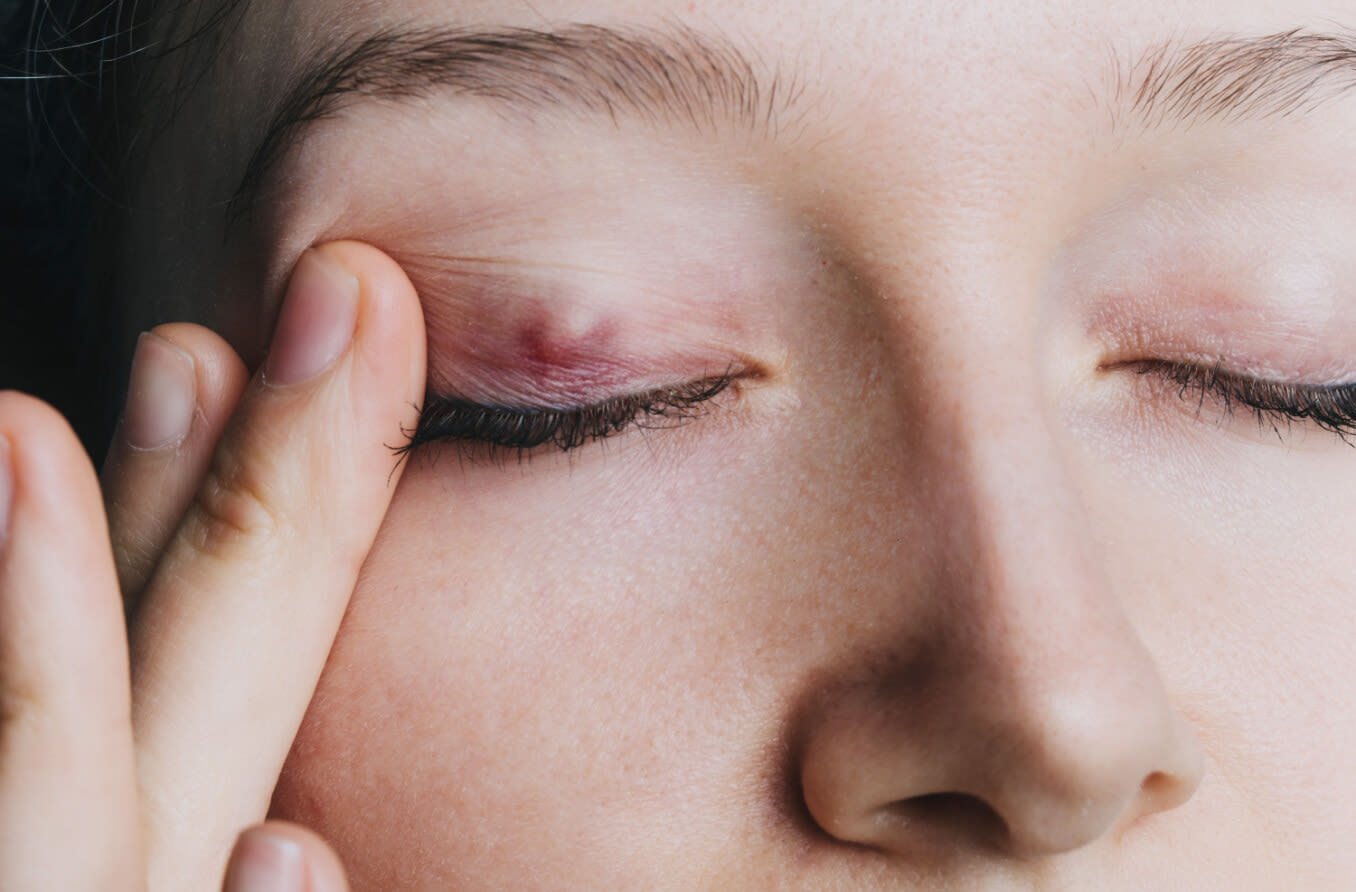This is a detailed close-up photo of a white woman's face, capturing her dark brown hair and neatly groomed, dark-colored eyebrows. The image focuses on her eyes, particularly highlighting her left eyelid. She is seen using her middle finger to pull back her left eyelid, revealing a prominent red bump, which resembles a barley eye or upper eyelid blepharoplasty. The bump appears painful and noticeable against her otherwise clear skin, which shows no visible signs of aging or wrinkles. Her fingernails are short, and she is wearing mascara on her lashes. The composition of the photo extends from just above her eyebrows to slightly below her nose, emphasizing the irritation on her eyelid while leaving her other eye and the rest of her face unblemished.